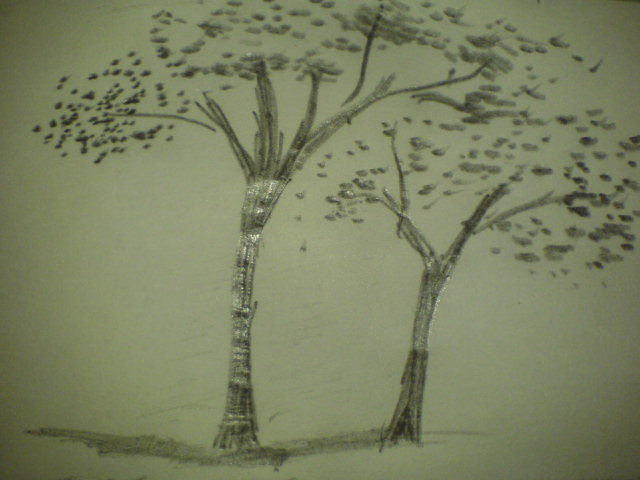This highly detailed pencil drawing features two trees on a pristine white sheet of paper. The trees are rendered with meticulous attention to detail, showcasing branches that shimmer with hints of silver. Beneath the trees, gentle shading suggests a grassy area, while circles filled in with care mimic the appearance of leaves. The leaves, though not directly connected to the branches, expand outward to fill the composition, with some appearing as though they are gracefully falling to the ground. 

The larger tree boasts seven branches, each elegantly extending from the robust trunk. In contrast, the smaller tree, positioned nearby, has four branches—two reaching to the left and two to the right. Beside the trunks of both trees, subtle pencil shading adds depth and dimension to the scene. The intricate combination of detailed branches, thoughtfully shaded grass, and artfully depicted leaves creates a captivating and serene landscape on paper.